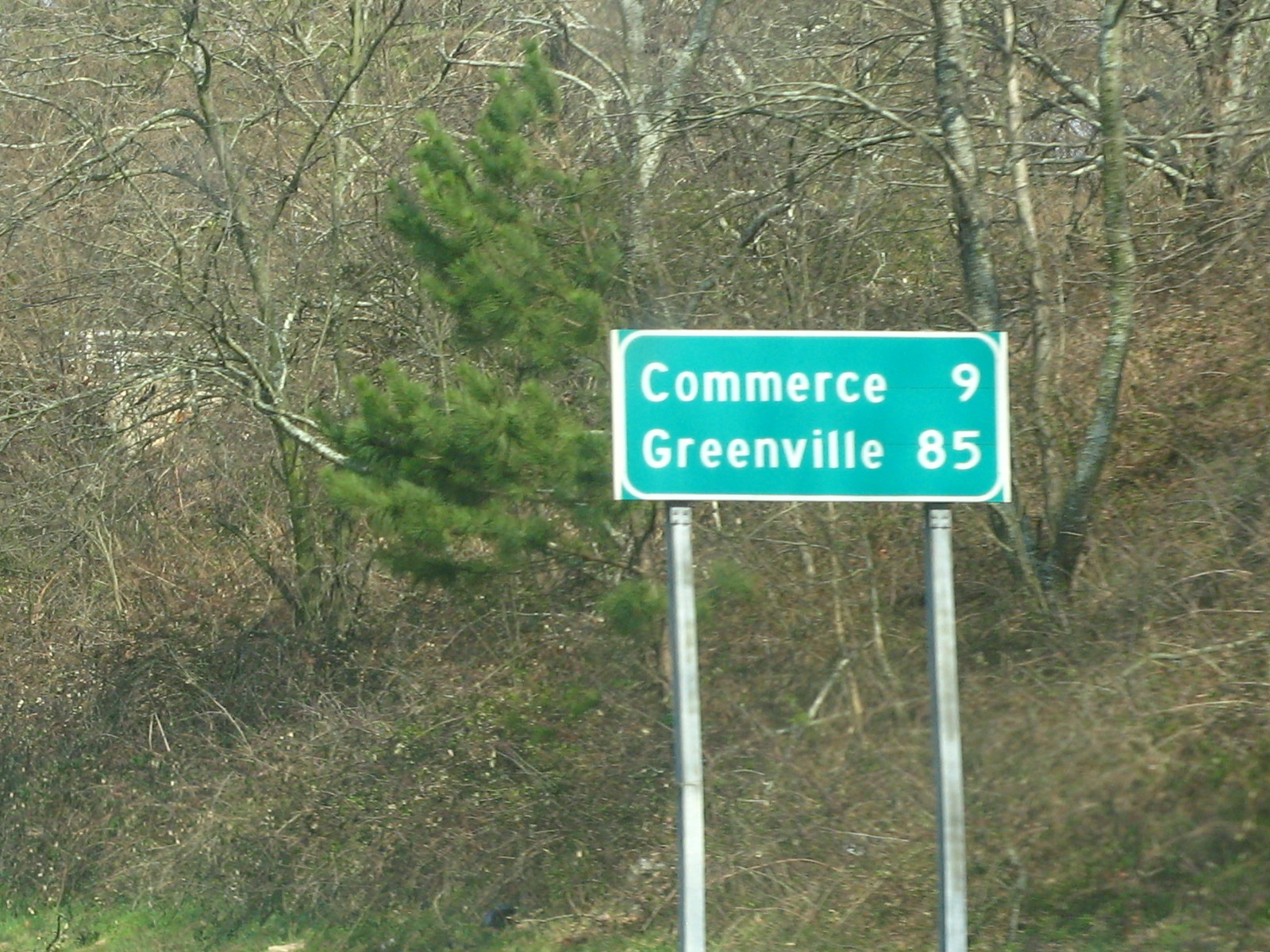This outdoor photograph captures a green street sign situated slightly to the right of the image, supported by two long silver poles. The sign, rectangular and landscape-oriented, appears slightly wider than it is tall. The poles, beginning from the bottom edge of the image, rise about halfway up, though their point of affixation is off-frame.

The sign itself is a light greenish-teal color with a white border. It features white lettering indicating two cities: "Commerce" with "9" miles and "Greenville" with "85" miles beneath it. The sign, seemingly disproportionate to the robust poles, conveys a sense of imbalance.

In the background, an upslope of a hill is densely populated with mostly leafless trees, save for one prominent evergreen with green needles. The ground is covered with brown grass and scattered sticks, contributing to a somewhat untamed appearance. The image was taken on a sunny day, casting natural light on the entire scene.